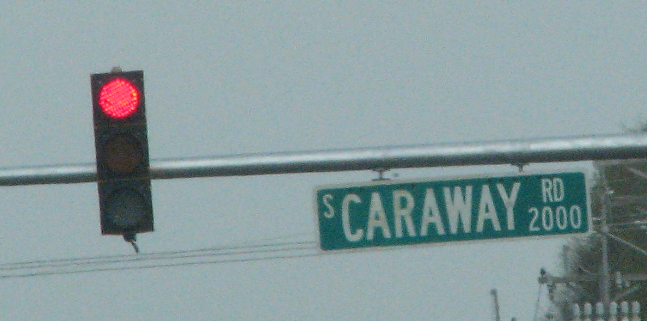The image captures a dreary scene dominated by an overcast, gray sky, emphasizing a foggy or cloudy atmosphere. At the center, a prominent silver metal pole extends horizontally across the frame. Attached to the pole on the left side is a black traffic light, currently illuminated in red at the very top, while the yellow and green lights remain off. 

To the right of the traffic light, hanging from the same pole, is a long rectangular green street sign with white borders. The sign reads "South Carraway Road," with "2000" indicating the street number. In smaller white letters, "S" appears at the top left corner, followed by "C-A-R-A-W-A-Y," "R-D," and "2-0-0-0" in smaller text beside and below the main name.

In the background, a network of power lines extends across the image from right to left, originating from what appears to be a telephone or electric pole, identified by its cylindrical attachments. Trees are faintly visible in the bottom right corner, adding to the overall somber and overcast ambiance.